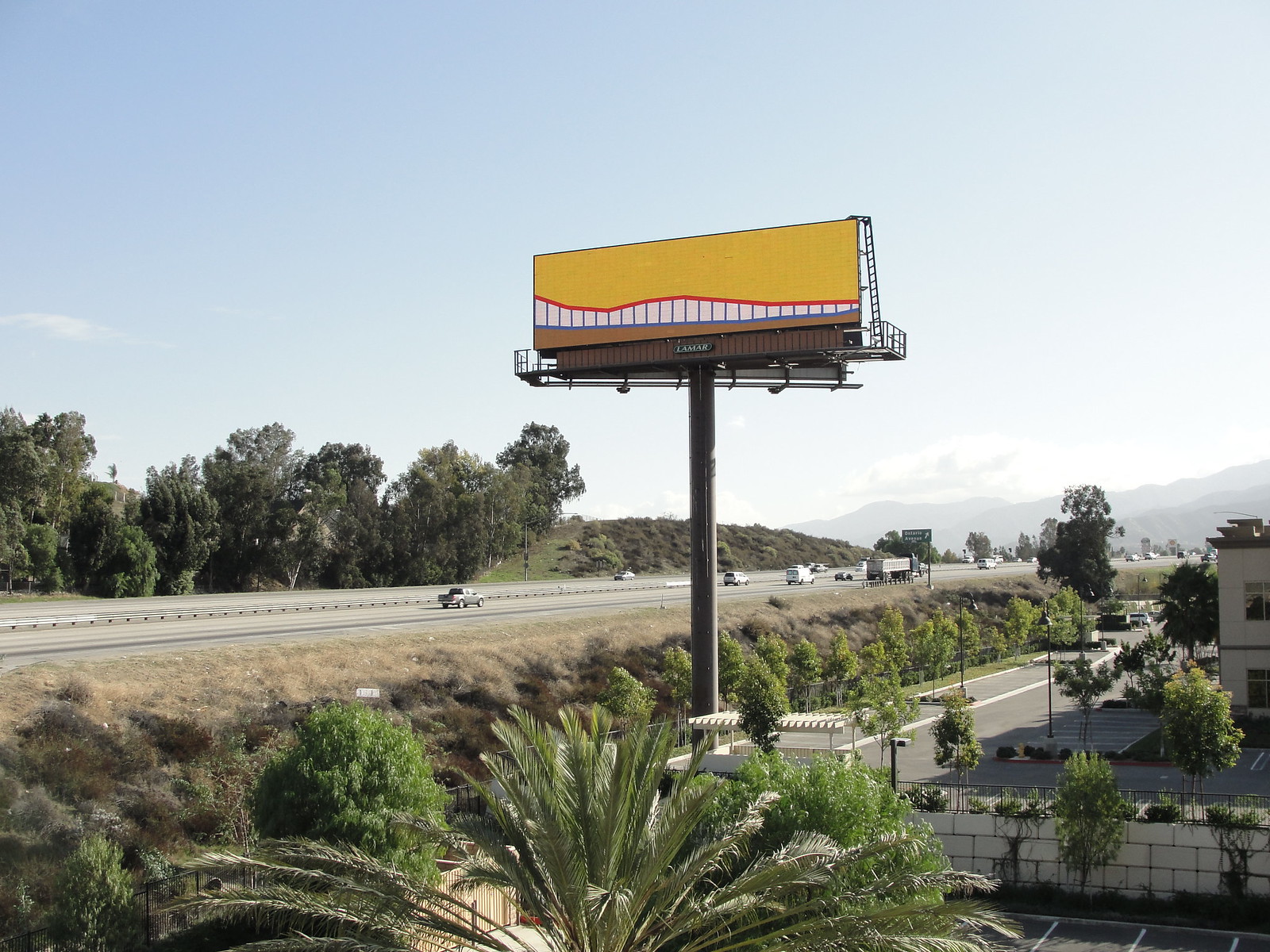The image depicts the early stages of a billboard's assembly. The billboard features a striking gold background with intricate artwork that resembles a roller coaster, its track vividly outlined in red. Beneath the primary display area, the name of the billboard is faintly visible, hinting at further details yet to be completed. An airborne scaffold is set up beside the billboard, with a ladder extending up to the top, providing workers access. On the left side, a walkway is discernible, likely for maintenance purposes.

The billboard itself is anchored by an exceptionally thick, brown pole that extends down into the parking lot of a nearby building. Below the scene, a busy freeway is captured, with cars travelling in both directions. In the background, a picturesque range of mountains rises, bordered by clusters of trees on either side of the image. The well-maintained parking lot beneath the billboard is divided by a white wall and flanked by a structure, adding to the urban landscape.